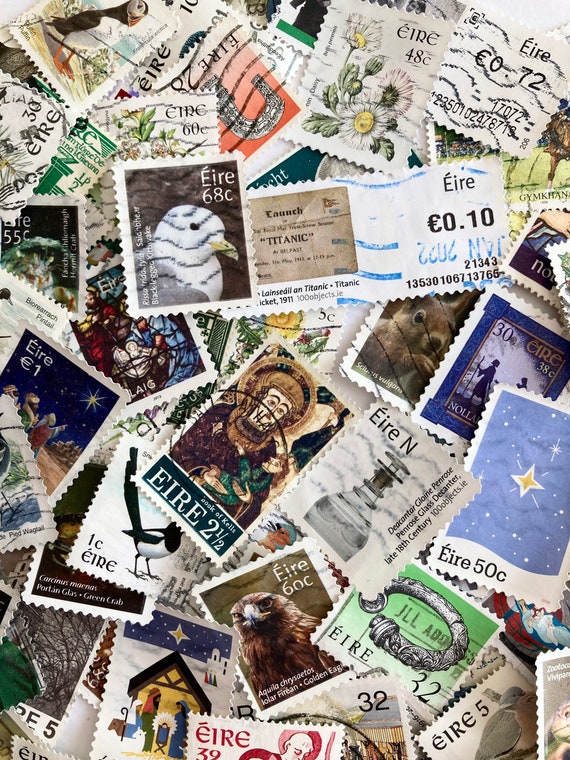This photograph showcases a scattered assortment of postage stamps laying on a table. The stamps, layered over each other, all bear the inscription "ÉIRE" and come in various denominations, ranging from 2.5 cents to 68 cents. Prominently, towards the top left of the image, there's a stamp featuring a pigeon marked with "ÉIRE 68c." Below this, at an angle, is a stamp with a monkey, labeled "ÉIRE 2.5c." Just beneath, a slanted stamp depicts a brown hawk, stamped with "ÉIRE 60c." Amongst the collection, other noticeable stamps include one with a magpie, another with a nativity manger scene, a white bird with a yellow beak, a puffin, and one adorned with white flowers, possibly daisies. The stamps showcase a variety of colors including blues, greens, oranges, reds, and pinks. Some stamps appear to have been used, as evidenced by black lines marking them. The varied and vibrant collection offers a detailed glimpse into the diversity of postage stamps marked with "ÉIRE."